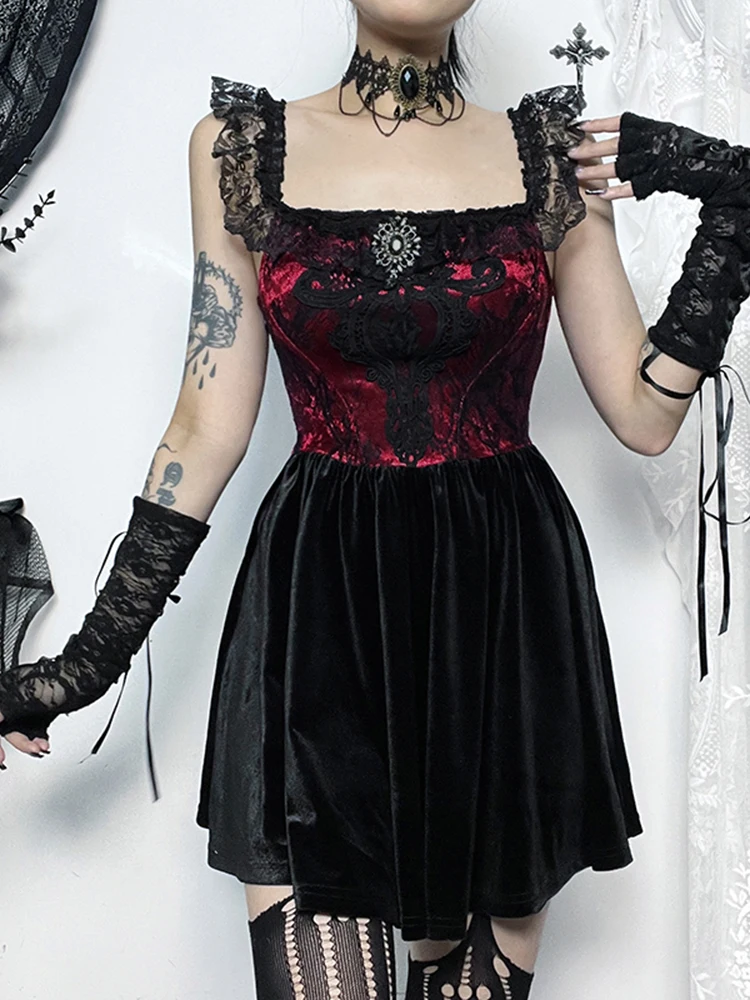A young woman stands in front of a white wall adorned with white lace and contrasted by black lace curtains in the upper corners. She is dressed in a goth outfit with intricate details. Her ensemble features a sleeveless top with black lace straps and a red bodice overlaid with black lace, accentuated by a black brooch at the chest. Around her neck, she wears a black lace choker with a large black brooch in the center. Her arms are covered in black lace gloves that extend almost to her elbows, secured with ties and adorned with ribbons. Below, she dons a black velvet skirt that flares slightly above her knees and pairs it with thigh-high tights intricately ripped in a vertical design. Her look is completed by visible tattoos on her left arm. The image is captured from just above her chin, leaving her face out of the frame, and presents a striking contrast between her dark attire and the light gray background with additional elements like a black hat hung on the left side of the wall.